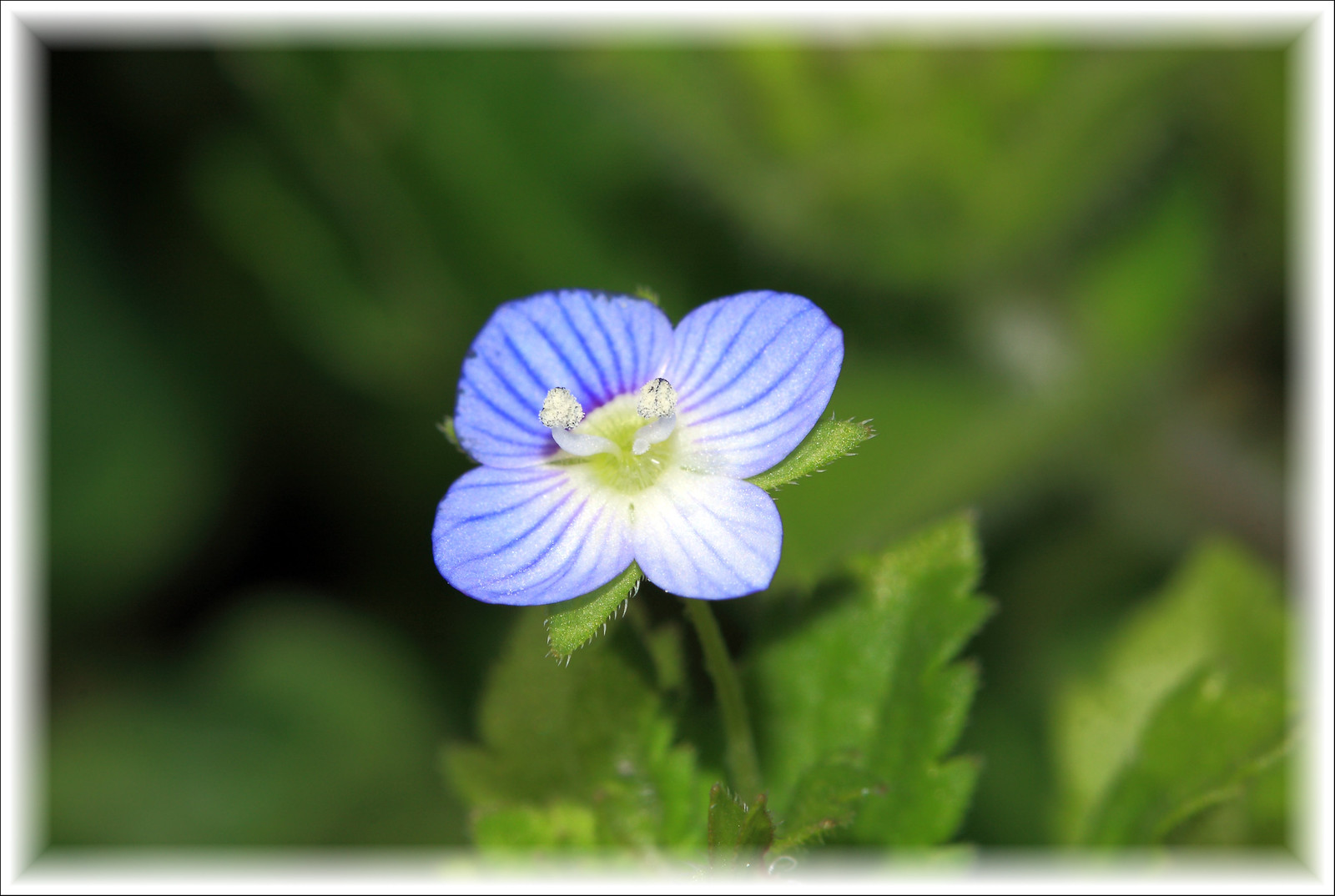This photograph, captured in natural daylight, features an extreme close-up of a delicate four-petaled flower. The image is framed with a thin black pinstripe border, followed by an inner beveled white border that gradually fades and blurs into the photo itself, creating a seamless transition. The background exhibits a bokeh effect with varying shades of out-of-focus green foliage and black, especially prominent in the upper left and right corners.

The central subject is a light purple flower, transitioning to almost white towards the center, adorned with dark purple veins that radiate outward from its lime green core. This center houses two stamens topped with light green puffs. Surrounding the flower and more defined in the lower right corner are green, slightly furry leaves attached to the same stem. The leaves, some triangular with small spokes, descend down the green stem, contributing to the natural, intricate look of the plant.